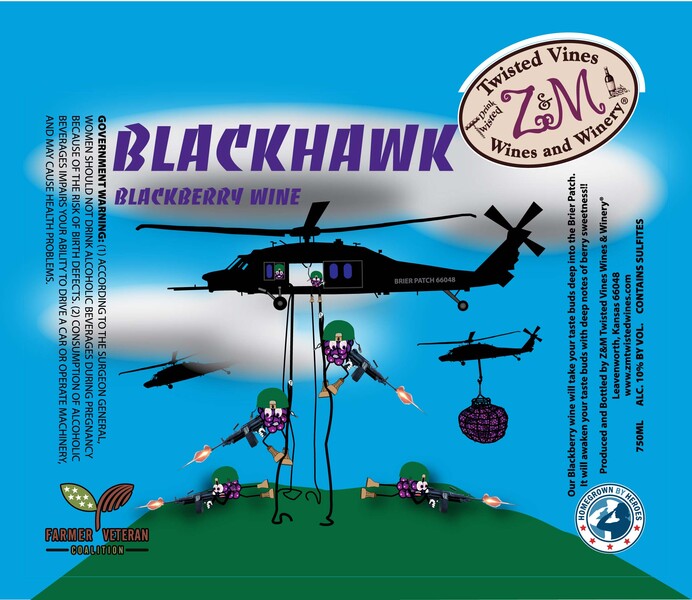This is a detailed cartoonish-style wine label for "Black Hawk Blackberry Wine" featuring a military theme. At the top, in bold purple text, is the name "Black Hawk Blackberry Wine". The sky is a bright blue with white clouds, partially obscuring another helicopter. In the center, a Blackhawk helicopter is seen with its side door open, revealing creatures resembling anthropomorphized bunches of grapes or California Raisins, wearing green helmets. Some of these grape soldiers are rappelling down to a green patch of lawn below, carrying and actively firing machine guns, with visible orange and yellow muzzle flashes. On the ground, more grape soldiers in green helmets and brown boots are positioned behind rocks, also firing their weapons. Additional helicopters are in the background, one carrying a large net full of grapes. The upper right-hand corner features a white oval logo with black and purple detailing that reads "Twisted Vines, Z&M Wines and Winery" along with a small image of a wine bottle and the tagline "Drink Twisted." At the bottom left, a circular logo says "Homegrown by Heroes," while the bottom right bears the "Farmer Veteran Coalition" emblem, featuring leaves. Both the left and right sides contain vertically aligned text with ingredients and a government warning about the alcohol content, 10% by volume, indicating it is a 750mL bottle containing sulfites. The imagery and text aim to create a unique and playful advertisement for the wine product.